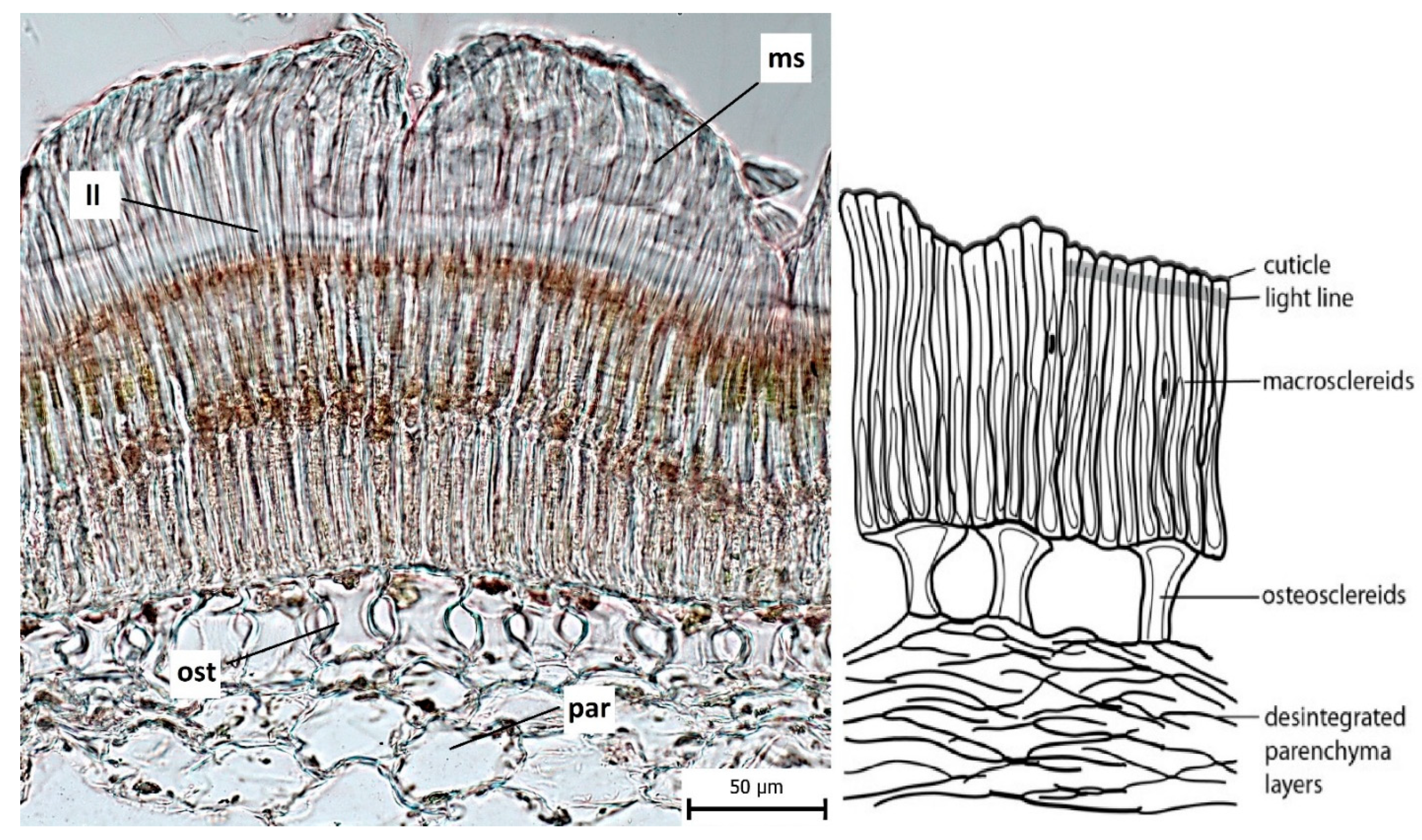This rectangular image presents two diagrams side by side, illustrating detailed microscopic views of what appears to be layers of either skin or a membrane. 

On the left side, the image features left-hand diagram with gray and brown striped sections representing the layers. The top layer is marked with the letters "MS" and has a line pointing downward towards the first layer, which has fine lines across it. An annotation labeled with "II" can be seen below this layer, presenting a reddish tint. More detailed structures are visible beneath this, marked as "OST" and "PAR," with rounded sections near the bottom. A scale marker labeled "50 UM" in the lower right corner indicates the magnification level of the image.

The right-side diagram is presented in black and white, serving as a more schematic representation of the layers shown on the left. The uppermost layer is labeled "cuticle light line," followed underneath by terms such as "macroscleroids" and "osteoscleroids," eventually leading down to "disintegrated parenchyma layers." This diagram clearly breaks down and labels the anatomical structure seen in the colored image, offering a detailed identification of each layer and its corresponding terminology.